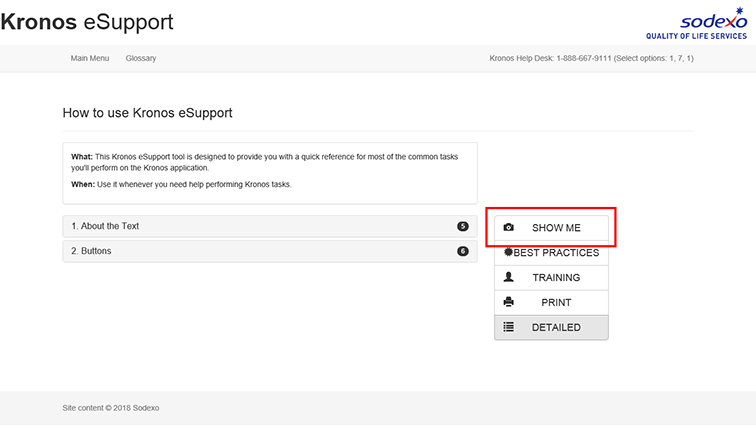The image depicts a comprehensive support screen for a website named Kronos eSupport. In the top left corner, "Kronos eSupport" is visible, denoting the platform being used, while the top right features the blue text "Sodexo Quality of Life Services," indicating the service provider.

The background of the screen is primarily light gray, creating a neutral canvas for the content. On the left side, there is a vertical sidebar with sections labeled "Main Menu" and "Glossary." Adjacent to this, within the same light gray background, the section titled "Kronos Helpdesk" is accompanied by a phone number, along with a prompt to select options number 171.

Further down, the screen provides instructions under the heading "How to Use Kronos eSupport." Below this, there are sections titled "What" and "When," each accompanied by descriptive text. Following these sections, two additional options are presented in light gray rectangular boxes: "About the Text" (labeled as number one) and "Buttons" (labeled as number two).

On the right side of the image, there is a list comprising five options: "Show Me" (highlighted with a red rectangle), "Best Practices," "Training," "Print," and "Detailed," with the last option highlighted in gray. This layout emphasizes interactive elements available to the user.

At the very bottom of the image, on a white background, the text "Site Content 2018 Sodexo" appears, signifying the date and ownership of the content. The entire interface combines structured navigation with helpful information to guide users through the Kronos eSupport platform effectively.